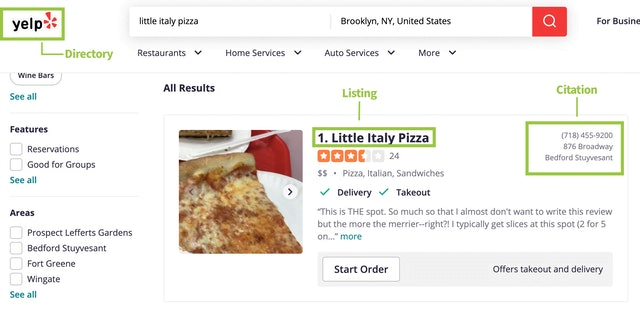The screenshot from the Yelp website prominently features the Yelp logo in the top left corner, displayed in a green box. The logo consists of the word "Yelp" in black letters, combined with an orange icon to its right. Directly beneath the logo, the word "Directory" is displayed, next to a search button. 

The main focus of the page is a listing for "Little Italy Pizza," located in Brooklyn, New York, United States. This is the top search result, marked as number one. The listing includes an image of a pizza and provides detailed information: a phone number and address, a price range starting at $2.00, and cuisine types listed as Pizza, Italian, and Sandwiches. The restaurant boasts a rating of three and a half stars, based on 24 reviews.

Additional icons indicate that the restaurant offers delivery and takeout services. A highlighted customer review reads, "This is the spot, so much so that I almost don't want to write this review but the more the merrier, right? I typically get slices at this spot, two for five on..." The full comment is truncated, suggesting more details are available. At the bottom of the listing, a prominent "Start Order" button encourages users to place an order directly through the website.